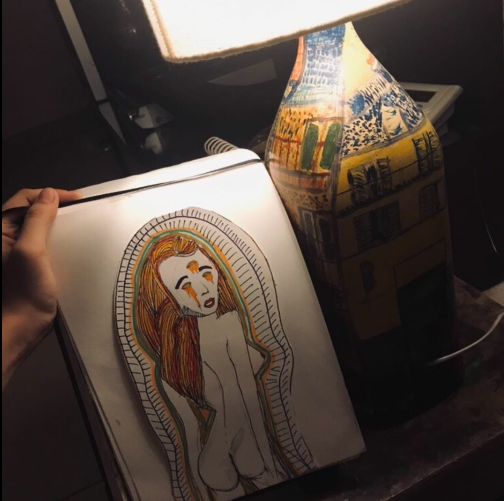A vibrant square image captures a person’s hand on the left side as they prop up a sketch pad on a table. The table itself supports a uniquely designed blue and yellow table lamp that emits a soft glow, illuminating the otherwise dim room. The centerpiece of the sketch pad is an artistic rendering of a woman with brown hair, undressed and viewed from behind yet slightly in profile. The sketch artfully details the top half of her body, cutting off at the legs, and is predominantly illustrated in brown hues accentuating her hair. The serene, artistic ambiance of the scene is accentuated by the minimalistic combination of light and shadow, focusing the viewer’s attention on the delicate sketch.